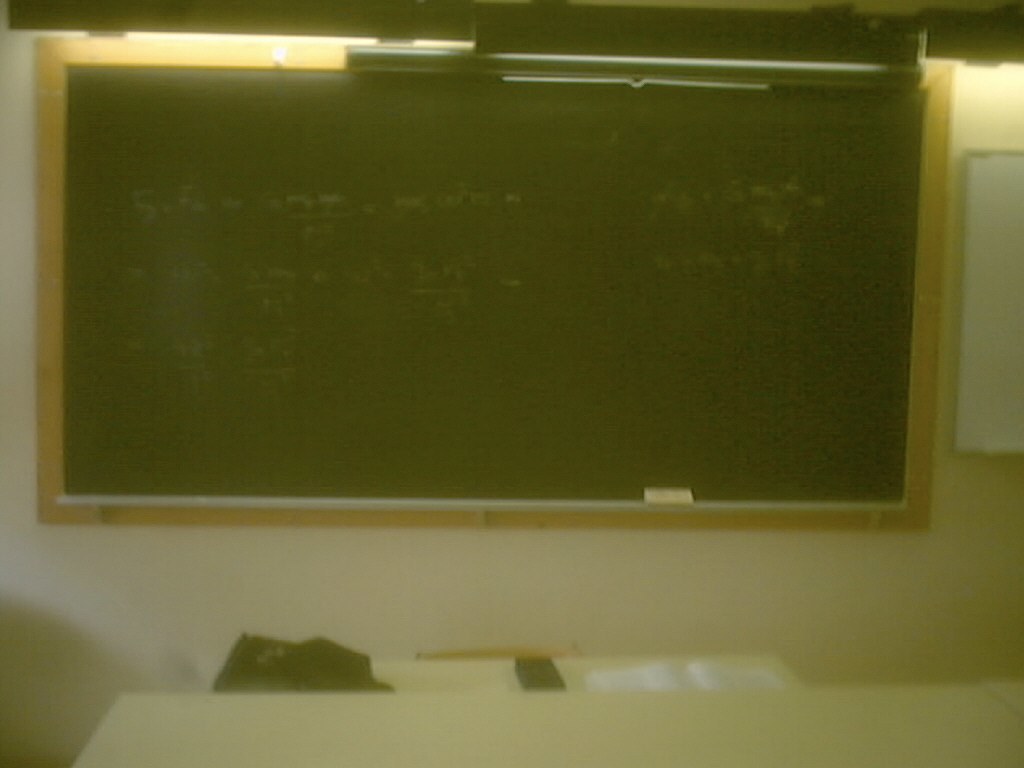The image depicts an old-fashioned classroom with a large black chalkboard framed in light wood taking up most of the background. Despite some faint, unreadable chalk writing, the board appears mostly clean. Above the chalkboard, a light shines down, illuminating the scene below. There's also a black casing, possibly the housing for a rolled-up projection screen. To the right of the chalkboard, partly visible, is a smaller whiteboard.

Beneath the chalkboard runs a long white desk, upon which an assortment of items rests. On the desk, there is an open white book or notebook, a black bag, and a smaller black rectangular object that looks somewhat like a remote. Along the bottom edge of the chalkboard is a narrow ledge where a rectangular white object, presumably an eraser, sits. In front of the white desk, there's a taller white surface, which might be another desk or a canvas. Everything appears slightly blurry, lending a nostalgic, old-time feel to the image.